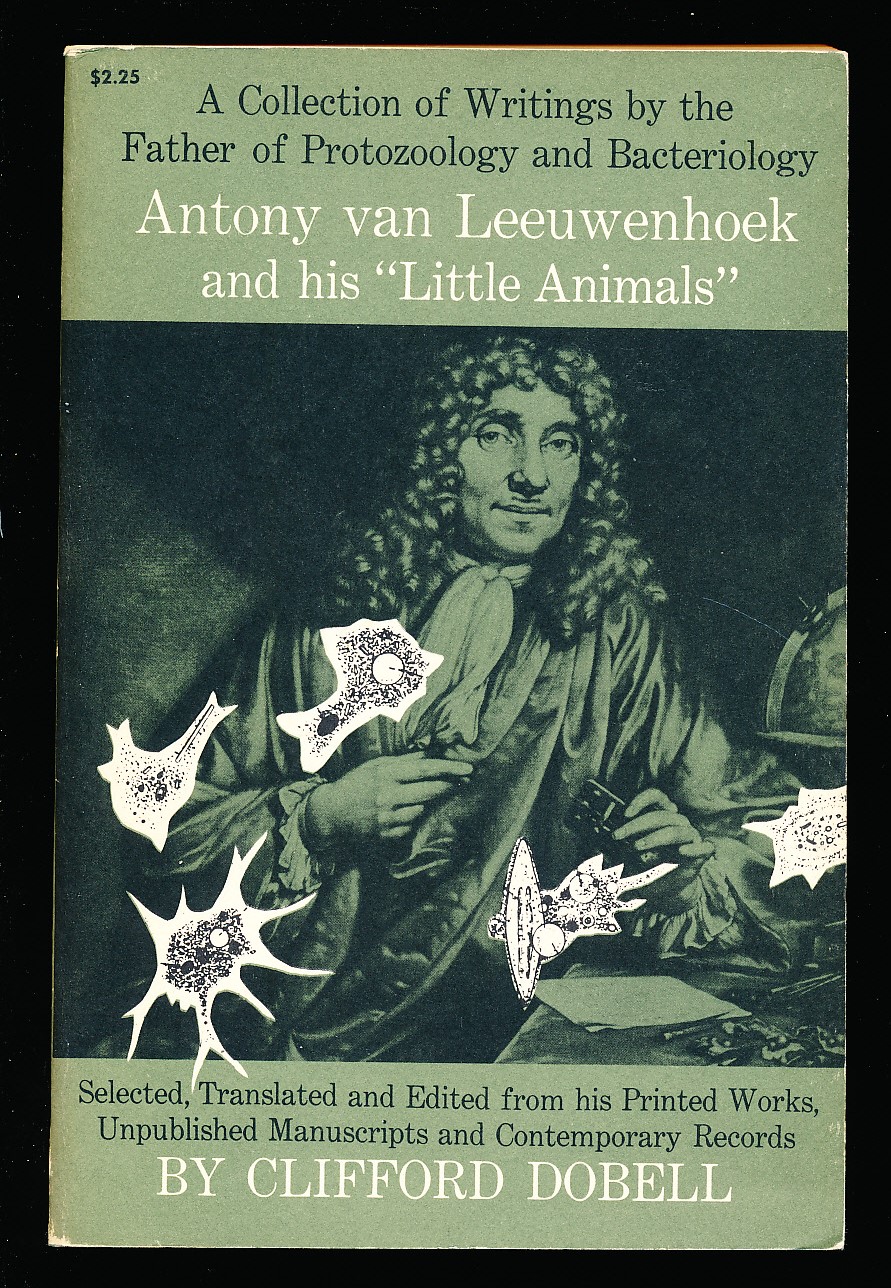This photograph showcases the cover of an old, well-worn book set against a completely black background. The book itself, tinged in a dull green, features prominently an illustration in the center, rendered in an old-fashioned printed style. The illustration depicts a man with a long curly wig, a flowing robe, and a white necktie, presumably signifying an 18th-century figure, likely Antony van Leeuwenhoek. Surrounding the central image are various cut-out designs resembling single-celled organisms, characterized by black dots on a white background.

At the top and bottom of the cover, olive green rectangles host important textual details. The top rectangle states in black text: "$2.25, a collection of writings by the father of protozoology and bacteriology." Beneath this, in white text, it further clarifies: "Antony van Leeuwenhoek and his little animals." At the bottom, in black text, it reads: "Selected, translated, and edited from his printed works, unpublished manuscripts, and contemporary records." Finally, a prominent caption in big white text displays: "By Clifford Dobell."

The overall aesthetic suggests a vintage, possibly mid-20th-century design, combining a sense of historical gravitas with scholarly precision.